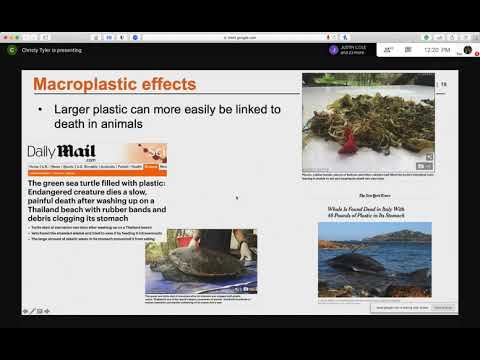The image appears to be a screenshot from a computer screen, showcasing a detailed and somber composition about the impacts of plastic pollution on marine life. At the top of the screenshot, a large black area dominates the header, followed by a gray section featuring a centered search bar. The predominant background color is black, making the central content stand out vividly.

In the middle of the screen, there is a large white area. The upper left corner features text in orange that reads "Macro Plastic Effects." Below this title is a black line separating it from the content underneath. The text following the line states, "Larger plastic can more easily be linked to death in animals."

To the right of this text, there is a small square image, presumably depicting a deceased animal. The image is somewhat vague, showing a cluster of brown fur with what seems to be a red tongue protruding from the middle, hinting at the gruesome reality of the subject matter.

On the left side, there is another section that resembles an excerpt from a news website. The header identifies it as coming from the "Daily Mail." The article headline is distressing and reads, "The green sea turtle filled with plastic, endangered creature dies a slow, painful death after washing up on a Thailand beach with rubber bands and debris clogging its stomach."

Below this news snippet, there is a square picture of a turtle, reinforcing the tragic subject of the article. In the bottom right corner of the screenshot, there is an image depicting what appears to be a body of water with a whale visible within it, likely serving as another tragic reminder of marine life affected by plastic pollution.

Overall, the screenshot is a poignant visual narrative that highlights the severe consequences of plastic waste on marine animals.